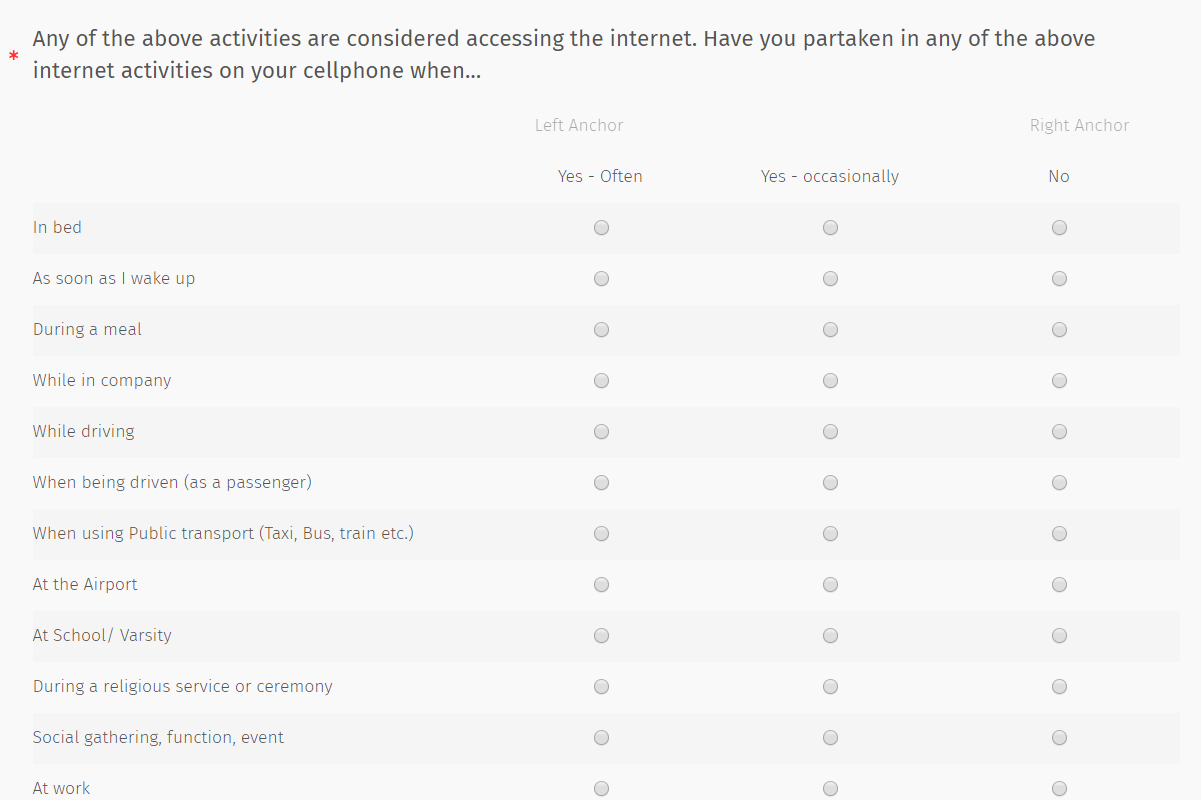**Descriptive Caption:**

The image depicts a screenshot of a questionnaire page with a light gray background. In the top left corner, there is a prominent, bright pink asterisk. To its right, there are two lines of medium-sized dark gray text that read: "Any of the above activities are considered accessing the internet. Have you partaken in any of the above internet activities on your cell phone? When?..."

Below this, a row of text is present, including two portions of small, light gray text — one centered reading "left anchor" and the other on the far right reading "right anchor." 

Further down, a line of text in slightly darker gray identifies the categories for the columns of radio buttons beneath it:
- "Yes - often" (first column)
- "Yes - occasionally" (second column)
- "No" (third column)

Following this, there are alternating rows of medium gray and light gray rectangles, each representing different scenarios in which the activities might take place. On the left side of each row, there is a title in light gray text, and beneath the column titles per row, there are light gray circular radio buttons with a medium gray outline and a subtle lighter gray shine on top.

The titles of each row, all left-justified, are listed from top to bottom as follows:
1. In bed, as soon as I wake up.
2. During a meal.
3. While in company.
4. While driving.
5. While being driven (as a passenger).
6. When using public transport (taxi, bus, train, etc.).
7. At the airport.
8. At school/varsity.
9. During a religious service or ceremony.
10. Social gathering/function/event.
11. At work.